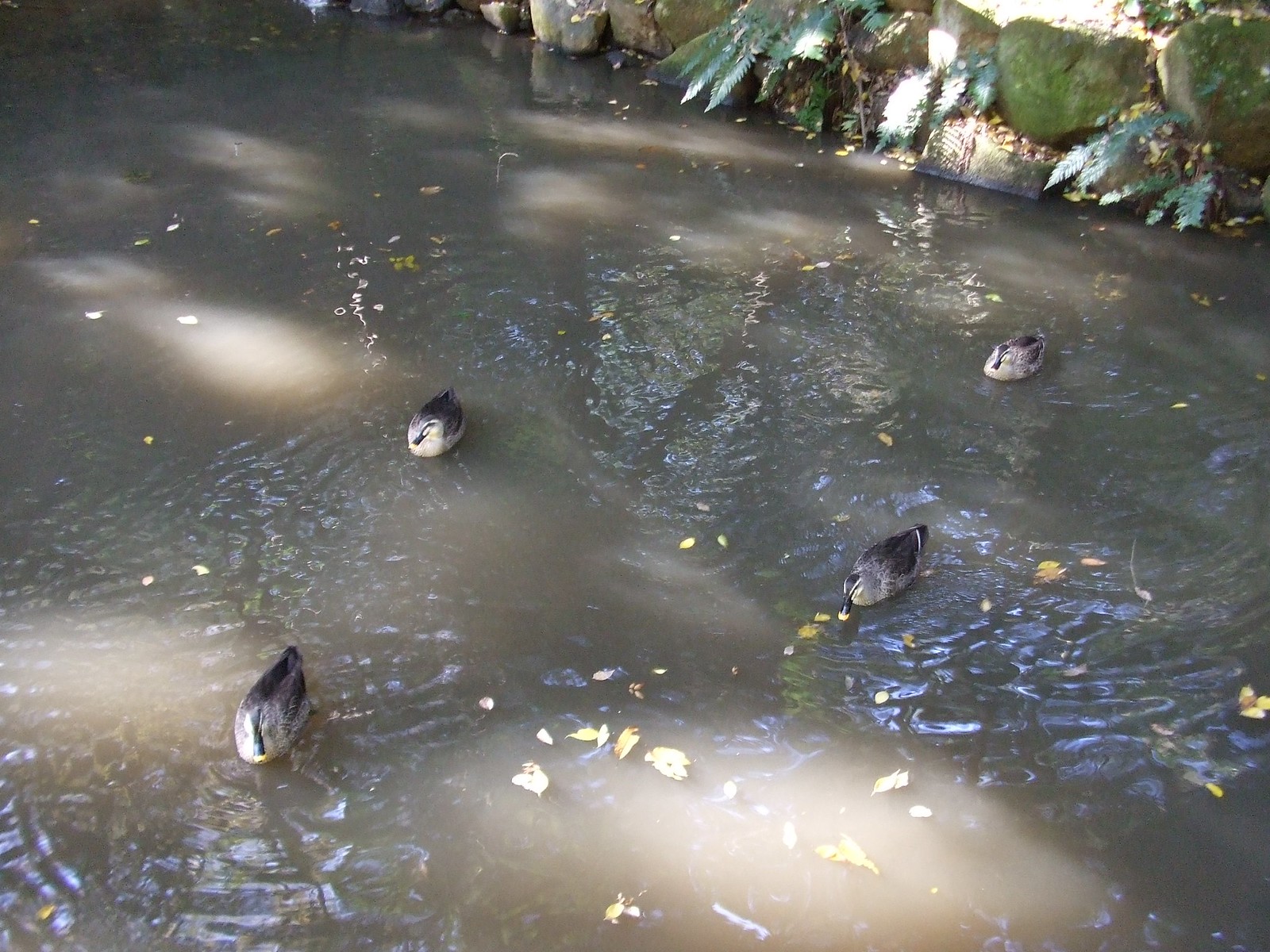The photograph captures a serene moment of four tan, female mallard ducks swimming in what appears to be a murky, dark gray pond. The water is still, faintly rippled, and dappled with sunlight that filters through overhead trees, creating bright spots and subtle color variations. The scene is decorated with dried fallen leaves floating on the water’s surface and broad green leaves reaching towards the pond from the top right corner of the image. Moss-covered rocks line the bank, suggesting a potentially man-made pond rather than a natural river or lake. One of the ducks can be seen with something in its beak, hinting at the possibility of people nearby tossing food. The ducks, with their dark bills and distinctive black eye stripes through white facial patches, are slightly spread out but seem to be swimming in the same general direction, adding a sense of purposeful movement to the tranquil setting.